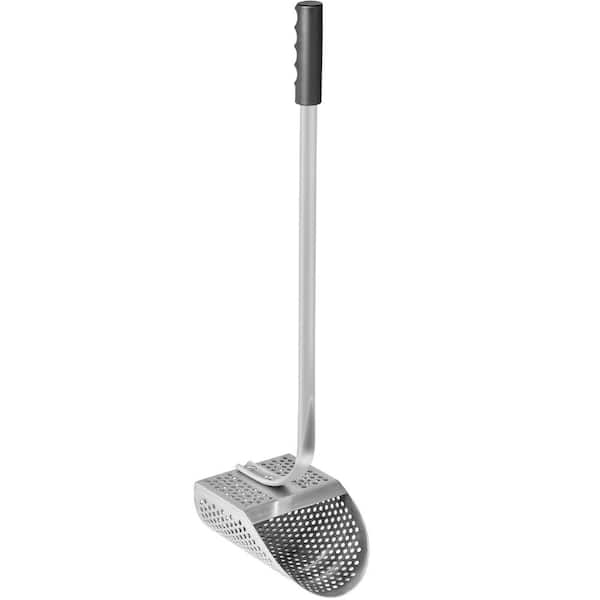The image depicts a stainless steel scooper with a long metal handle, designed specifically for sifting through sand, typically used by metal detector enthusiasts. The handle, extending up to a couple of feet long, features a black plastic or rubber grip with finger grooves for added comfort and control. It seamlessly bends and flattens out at the end to attach to a metal scoop. This scoop resembles a basket with numerous holes, ideal for efficiently sifting and filtering out unwanted debris. The product is showcased on a white background, emphasizing its sleek, all-metal construction and functional design.